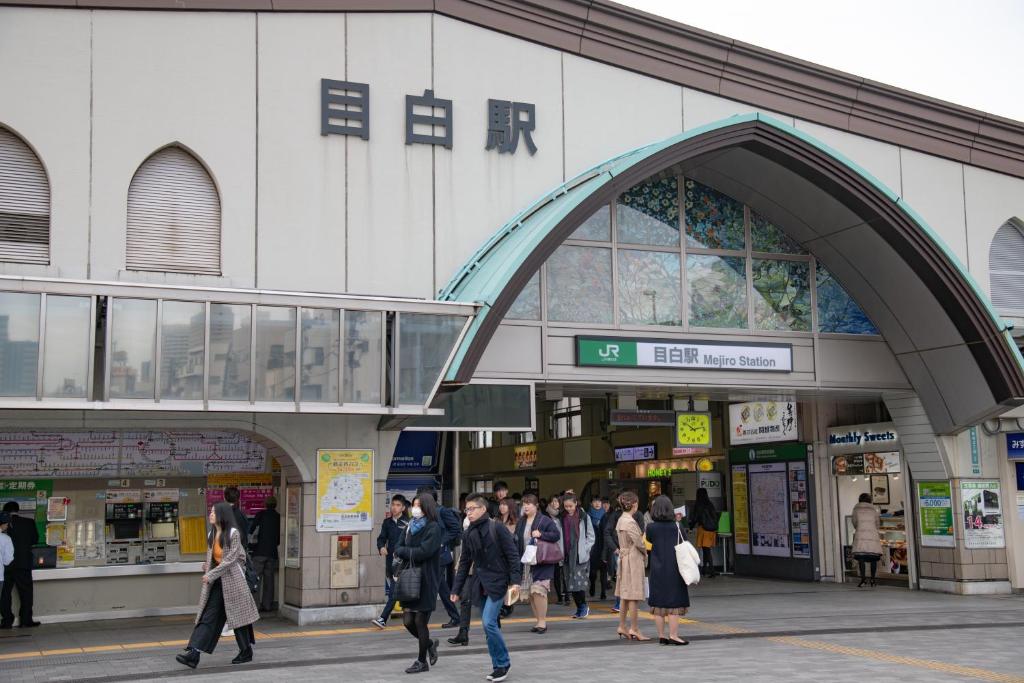A bustling scene unfolds just outside the entryway of a prominent building, capturing a snapshot of daily urban life. In the foreground, a light gray pavement is marked by two distinct yellow lines: one running horizontally on the left and another running vertically on the right. Approximately ten individuals are depicted walking out of the entrance, veering to their left. The imposing structure itself is predominantly gray, featuring a towering design that draws the eye upwards. 

A distinctive blue and gray hooded overhang can be seen above the entrance, providing a sense of shelter and architectural interest. Further up, the building transitions to a lighter shade of gray and proudly displays three dark gray Asian symbols, imparting cultural significance. Crowning the top of the building is a brown segment that adds a contrasting element to its facade.

Prominently displayed is a green and white sign that reads "Mijiro Station," indicating the building's use as a transportation hub. The very top right corner of the image offers a glimpse of the sky, rendered in a stark white that emphasizes the urban setting.